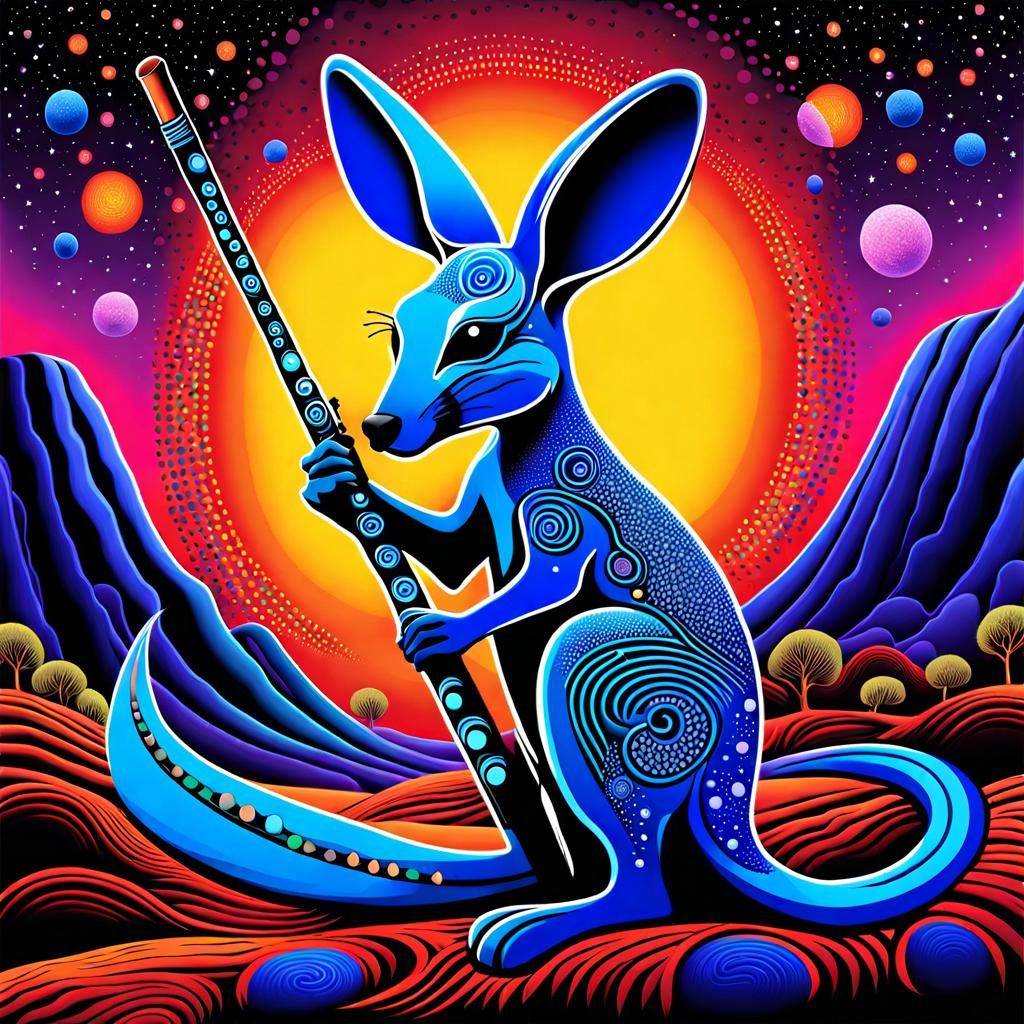The image portrays a highly stylized, psychedelic painting of a blue wallaby or baby kangaroo, possibly AI-generated or digitally created. The central figure of the blue wallaby features a swirling design that dominates its body, adorned with dots, lines, and circles, and boasts a black tummy. It holds a black stick or wand decorated with swirls and blue circles, ending in a red tip, in both hands. The scene unfolds with the wallaby standing on wavy ground resembling red spaghetti interspersed with blue balls. Surrounding the wallaby are floating multicolored balls, suggestive of a cosmic or space-like setting. Behind it, a gigantic sun with a yellow core and a red ring illuminates the background, which also includes stylized green trees and synthetic ocean waves, evoking a surreal and vibrant atmosphere.